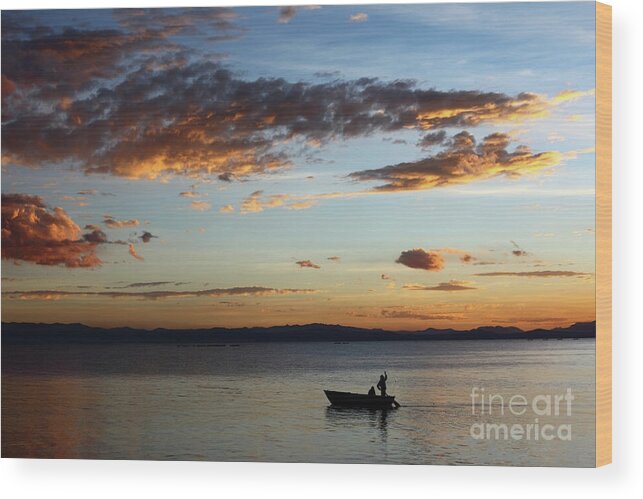This is a detailed photograph of a canvas, which appears to be framed with a wooden texture and a brown border, visible on the right-hand side. The canvas features a tranquil lake in the lower portion, with a calm body of water that subtly reflects the vibrant colors of the sunset. In the foreground, a small silhouette of a rowboat is occupied by two people, one sitting and one standing with a hand raised. The boat and its passengers are entirely black silhouettes against the water. The horizon is defined by a low mountain ridge also in silhouette, which adds depth to the composition.

Above the silhouette, the sky dominates the majority of the canvas and is filled with cotton ball-like clouds. These clouds reflect the descending sun, creating a gradient of colors from light blue at the top to warm oranges and yellows nearer to the horizon, blending beautifully into the scene. This illumination suggests the sun is setting on the right side of the frame, casting its final light and coloring portions of the clouds.

The photograph on the canvas is marked in the bottom right corner with the watermark "Fine Art America." The overall scene captures a serene and picturesque moment of sunset over a peaceful lake, with mountains in the distance and a blending of natural colors, emphasizing the gentle transition from day to night.